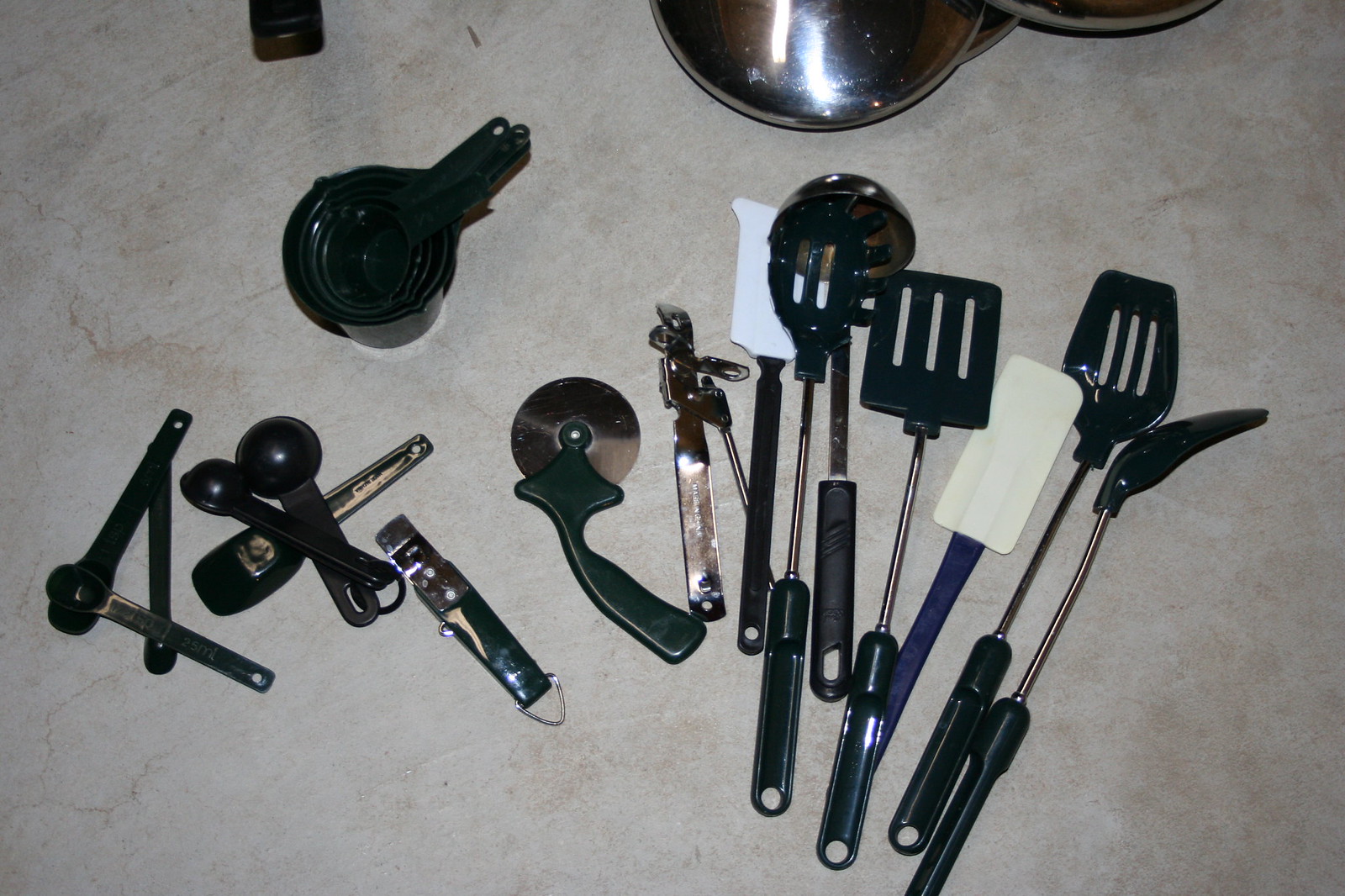This photograph captures an assortment of kitchen utensils sprawled across a tan marble countertop that features light brown accents. The utensils seem to be primarily made of metal and black plastic, with some colorful exceptions. Among them, there is a black spatula with a silver center handle, a pasta server stained with red sauce, and a soup ladle containing red soup. To the left side, an old-style silver can opener and a pizza cutter with a dark green handle are positioned next to an antiquated bottle opener with a green handle and silver top. The image also displays black measuring spoons and stacked black measuring cups, as well as two rubber spatulas—one with a black handle and white head and another with a dark blue handle and tan head. The backdrop of these utensils includes partially visible silver bowls, and all items are laid out in a seemingly disorganized manner.